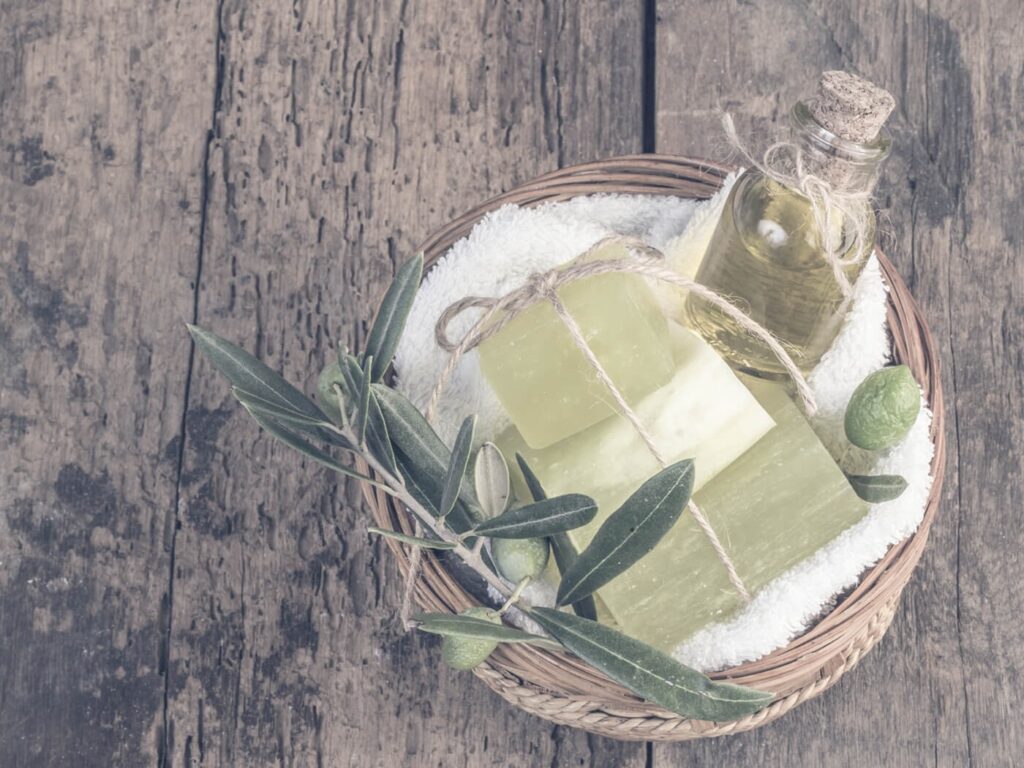The image captures an overhead view of a scene set on a medium brown, natural wooden table. At the center, slightly to the right, sits a round, natural wooden weave basket. The basket contains a pristine white terrycloth towel at the bottom. Resting atop the towel are three handmade bars of soap in varying shades of green—a light green, a milky white, and a darker green—each tied together with natural-colored string. In the basket, there is also a glass bottle filled with a greenish liquid, resembling olive oil or perhaps perfume, sealed with a cork and adorned with a bow made of the same natural-colored twine. Accompanying these items are a sprig of greenery with small green olives and a lone green olive laying inside the basket. The detailed and rustic presentation suggests a natural, handcrafted theme throughout the image.